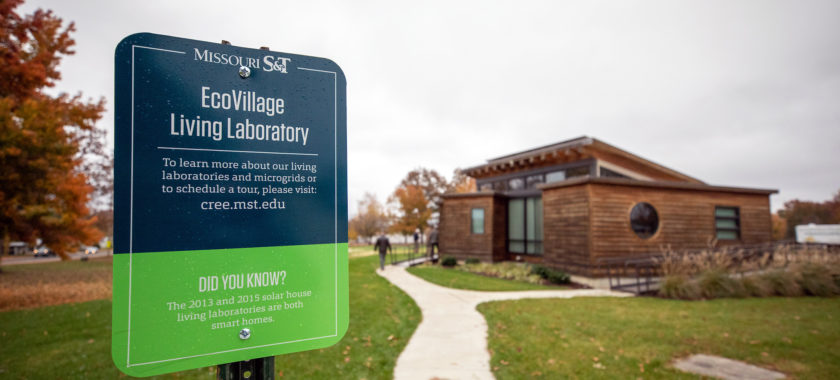This wide-angle photograph captures the Missouri S&T EcoVillage Living Laboratory, prominently featuring a blue and green sign in the foreground. The sign reads "Missouri S&T EcoVillage Living Laboratory" in white font. Below it, additional information directs visitors to cree.mst.edu for more details on the living laboratories and microgrids, and to schedule a tour. It also points out that the 2013 and 2015 Solar House Living Laboratories are both smart homes. The sign is secured with two silver bolts, and the bottom part says, "Did You Know?" followed by more white text. In focus to the left, you can see another part of the message, "Did you know the 2013 and 2015 Solar House Living Laboratories are both smart homes?"

In the background, the EcoVillage Living Laboratory features a modern wood-paneled house with a distinct circular window on the right, long paneled glass windows in the center, and a unique sloped roof likely designed for solar panels. The structure is surrounded by thoughtfully designed landscaping and a grassy area with a walkway leading to the house. A man stands on the walkway in the distance. The background is also adorned with two trees, one positioned to the far left of the sign and another in the center of the photo, adding a touch of nature to this innovative and sustainable living space.